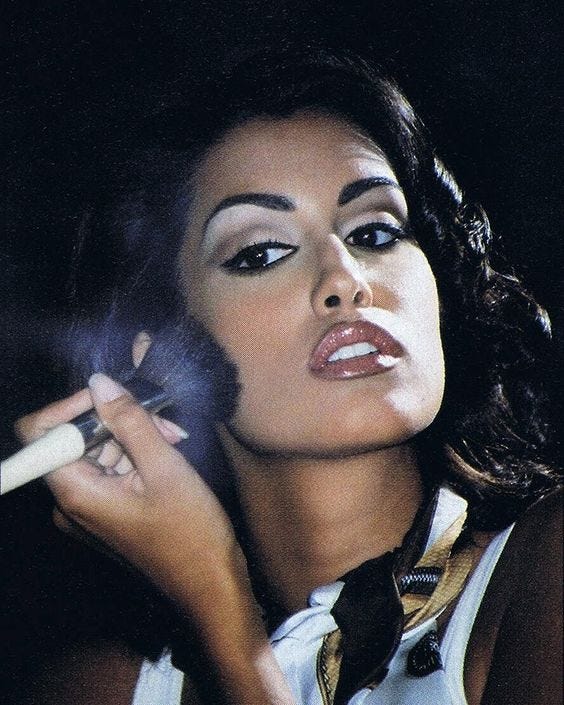The full-color image appears to be a glamour shot from the 1960s or a screenshot from an older movie. It features a strikingly beautiful young woman, possibly of Middle Eastern descent, with long, curled dark hair. Her makeup is meticulously applied, with dark eyebrows, black eyeliner accentuating her dark eyes, light eyeshadow, and glossy plump red lips. She is seen applying makeup to her right cheek using a brush held in her left hand, with a faint puff of powder visible around the brush. She seems to be gazing into a mirror, likely off to the left, based on her eye direction. The woman is dressed in a white top with a scarf tied around her neck in a neat knot, the scarf being white with gold and black accents, and she appears to have black sleeves. The background is black, enhancing the focus on her and adding to the overall elegance of the image.